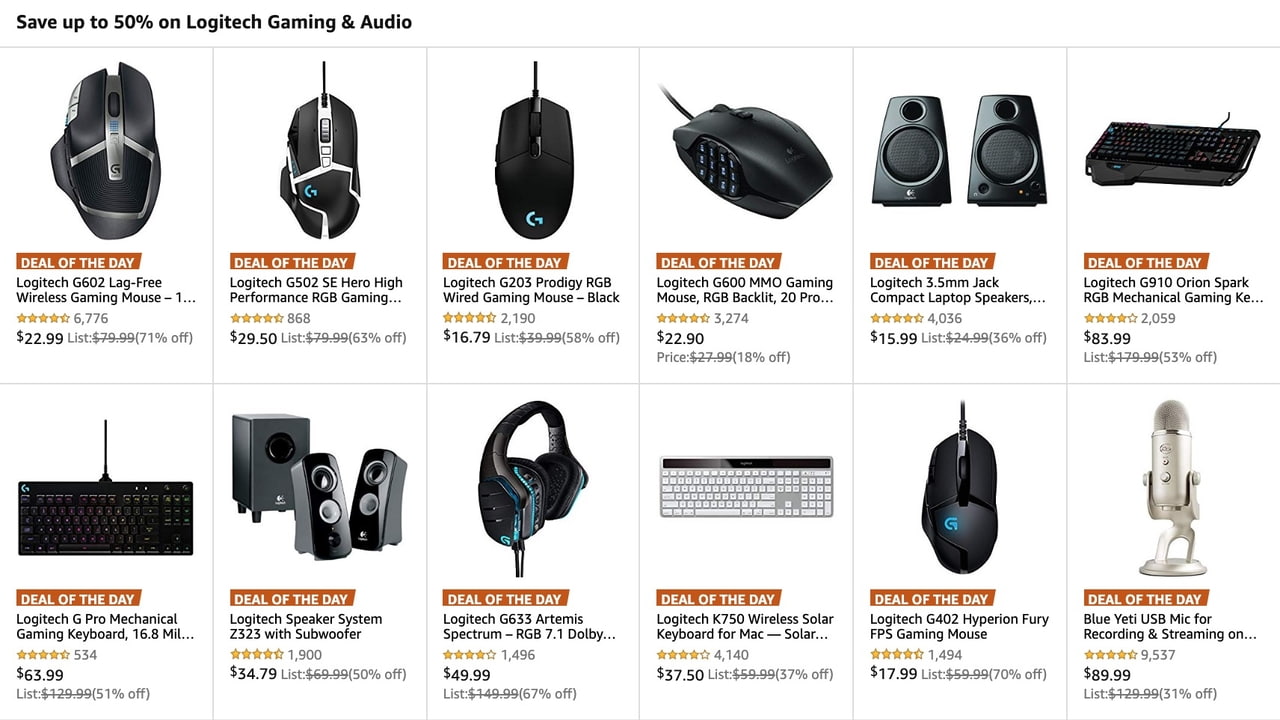This image showcases a promotional advertisement featuring two rows of Logitech products arranged from left to right, all highlighted with deals of the day. A banner at the top left corner announces "Save up to 50% on Logitech Gaming and Audio," catching the viewer's attention with its attractive savings offer.

In the top row, six products are listed, each marked with a "Deal for the Day" badge in a brown highlight with white text. The products and their prices are as follows:
1. A computer mouse priced at $22.99.
2. A computer mouse priced at $29.50.
3. A computer mouse priced at $16.79.
4. Another computer mouse priced at $22.90.
5. Logitech speakers priced at $15.99.
6. A Logitech keyboard priced at $83.99.

The bottom row continues with the following products:
1. A Logitech keyboard priced at $63.99.
2. A three-piece speaker setup priced at $34.79.
3. Over-the-ear headphones priced at $49.99.
4. A gray keyboard priced at $37.50.
5. A computer mouse priced at $17.99.
6. A silver microphone priced at $89.99.

All the products are displayed on a clean white background, enhancing the clarity and focus on each item and their respective details, such as name, reviews, and prices.